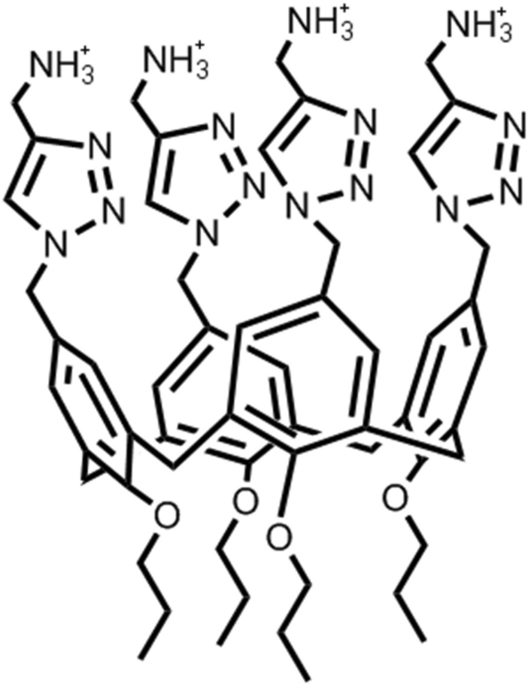The image is a detailed, black-and-white infographic of a molecular structure, drawn using computer software. It prominently features multiple representations of NH3 (ammonia) molecules interconnected by various chemical bonds. The structure consists mainly of nitrogen atoms (N) bonded to three hydrogen atoms (H) in the NH3 configuration. Every NH3 molecule is depicted with clear lines illustrating the covalent bonds between the atoms. Additionally, the diagram shows other chemical elements and compounds, though the primary focus remains on nitrogen and hydrogen bonds. At the bottom of the image, there are geometrical patterns, specifically four six-sided figures (possibly representing oxygen or another molecules), which are intricately connected to the NH3 structures. The background of the image is plain white, emphasizing the complexity and detail of the molecular bonds. Overall, the infographic aims to visually represent the compound structures and the relationships between different molecules.